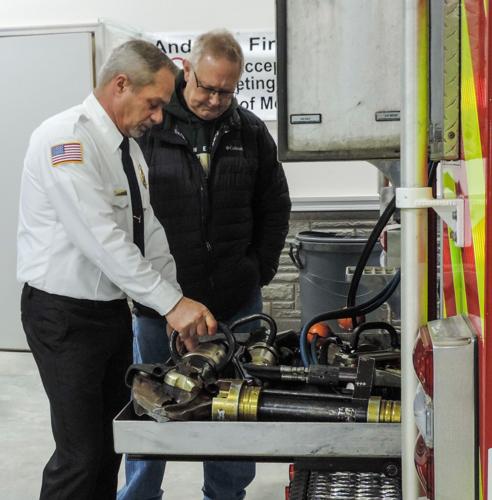In an indoor setting resembling a firehouse, two older men are captured examining firefighting equipment atop a platform. On the left, a man dressed in a white, button-down shirt with a black tie, black pants, and an American flag patch on his shoulder is seen holding an oxygen tank. Next to him on the right is a man in a black jacket, wearing glasses. Both are focused intently on the equipment before them. The room features white stone walls, a grey door in the top left corner, and a small sign with partially obscured black text. The colors in the scene include beige, tan, white, black, goldish yellow, orange, dark gray, yellow, and red, with a part of the wall reflecting these colors. A trash bin is positioned in the middle right, completing the detailed composition of the scene.